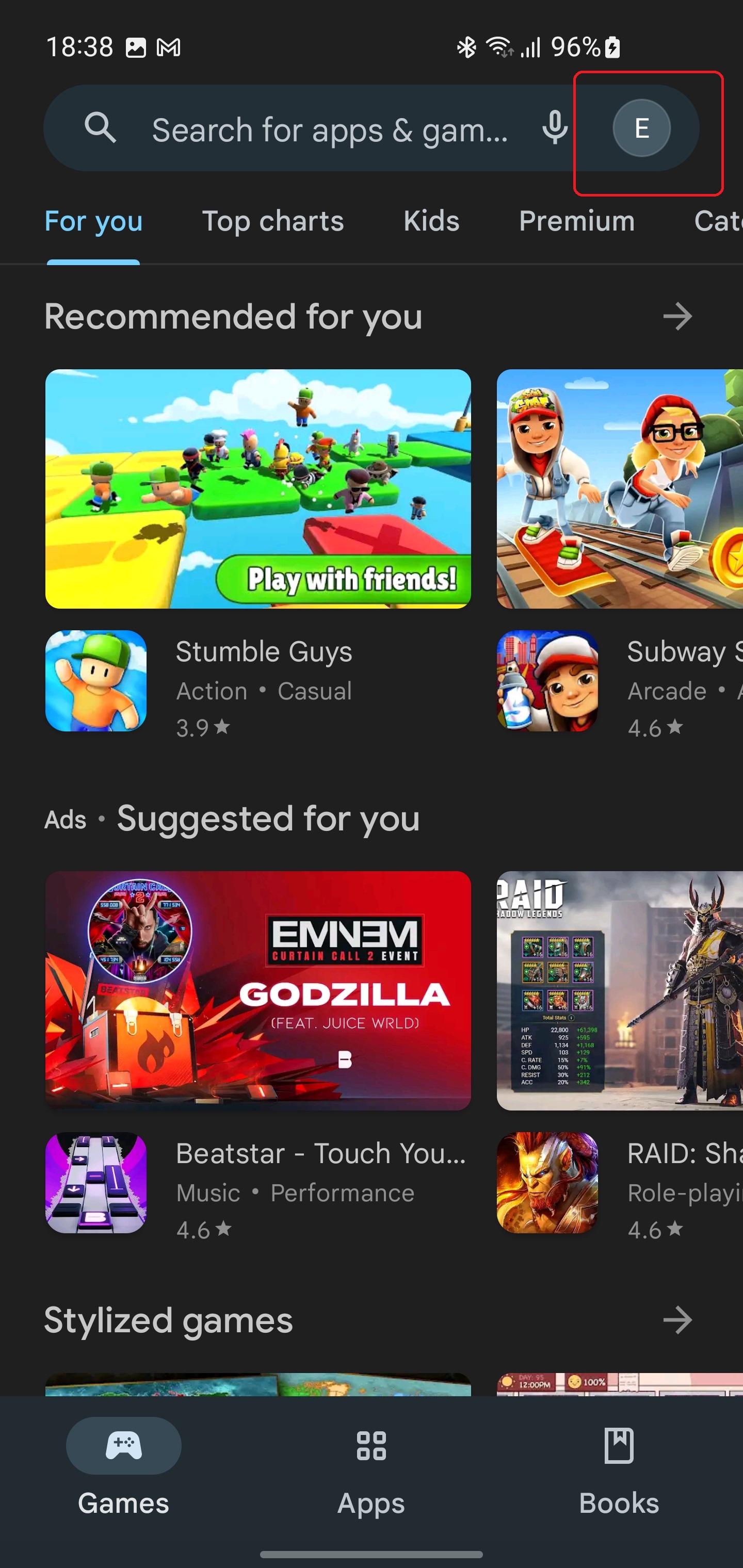The image depicts the home screen of the Google Play Store, shown in night mode with a black background. The interface primarily features three tabs at the bottom: 'Games,' 'Apps,' and 'Books,' confirming it is indeed the Google Play Store. The selected tab is 'Games,' which showcases six game suggestions as follows:

1. **Recommended for You:**
   - **Stumble Guys**: A casual action game with a rating of 3.9 stars.
   - **Subway Surfers**: An arcade game with a rating of 4.6 stars.

2. **Suggested for You (Ads):**
   - **Godzilla Music Game (possibly Beat Star)**: A music performance game.
   - **Raid Shadow Legends**: A role-playing game.

Below these, the heading "Stylized Games" is visible, though the specific games under this section are not shown.

At the top of the screen, there is a search bar. The status icons and indicators reveal that the device is connected to Wi-Fi, has full cellular signal bars, is showing a battery level of 96% with the charging icon active, and displays the current time as 18:38 (military or European time format). Additionally, there is a small user profile picture located in the upper-left corner of the screen.